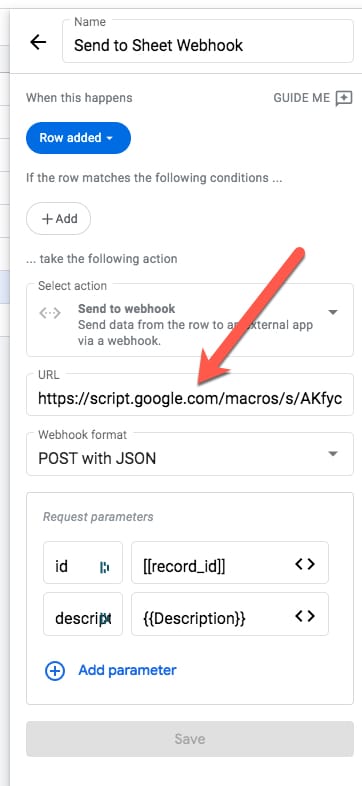**Caption:**

The image depicts a partial screenshot resembling the width of a smartphone screen. At the top, there's a header section with bold black text reading "Send to Sheet Webhook," accompanied by a left-pointing arrow on the far left of the same line. Just below this header, the phrase "When this happens" is followed by a horizontal blue oval containing white text that reads "Row added," featuring a small arrow pointing downward.

The next section of the screen states, "If the row matches the following conditions," providing options to take subsequent actions. A URL in its own tab starts with "https://script.google.com/macro/s/AKFYC," highlighted by a large orange arrow pointing towards it.

Beneath the URL, another section labeled "Webhook format POST with JSON" is visible. Below this, the "Request parameters" are highlighted in black, accompanied by a blue circle with a plus symbol inside and the text "Add parameter" next to it. Finally, at the very bottom of the page, there is a gray box with an option to save the configurations.